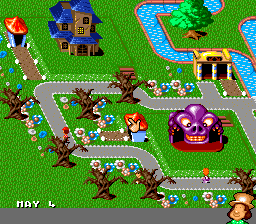The image is a small, pixelated, square screen from an older-style handheld or flash video game, reminiscent of Gameboy graphics. The scene depicts a quaint, cartoonish neighborhood with a central gray road winding through it, surrounded by various structures and features. A two-story wooden home with a blue roof and a sizable green yard stands out. Adjacent to the home is a garage topped with a red roof and what appears to be a coliseum-like building. 

In the lower right corner of the image, there is a large, friendly-looking purple creature next to a smaller creature with a red head and a blue body. The center of the town is dotted with several brown, somewhat spooky trees. To the top right, a river flows behind a structure resembling a car wash, creating a whimsical scene. Additionally, there is a small creek with a bridge running through the town. The top left features a haunted house-like structure, adding a playful spooky element to the otherwise cheerful village.